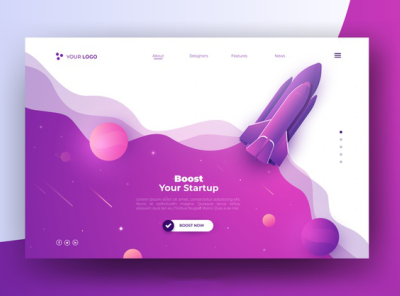The image depicts a website with a dual-colored background, primarily featuring vibrant shades of purple, pink, and white. The top half of the background is white, while the bottom half transitions to a rich purple.

In the upper left corner, a logo comprising three interlocking circles is displayed alongside the text "Your Logo". Positioned to the right of the logo are four navigation headers, culminating with a hamburger menu at the far right edge.

Centrally, the focal point of the website is an illustration of a spaceship angled diagonally towards the upper right. It navigates through a cosmic scene with a variety of planets: a prominent pink planet, a slightly larger purple planet, and two smaller pink planets, adding depth and intrigue to the visual.

At the heart of this space-themed design, white text stands out against the background, proclaiming "Boost Your Startup". Beneath this main headline, three lines of smaller text provide additional context. Directly below this section, a checkmark icon and text "Boost Now" serve as a call-to-action button.

The background of the overall website image contrasts with the website itself, showcasing a split of white on the upper portion and purple on the lower half. The design features considerable white space above the "Boost Your Startup" text, contributing to a clean and open layout.